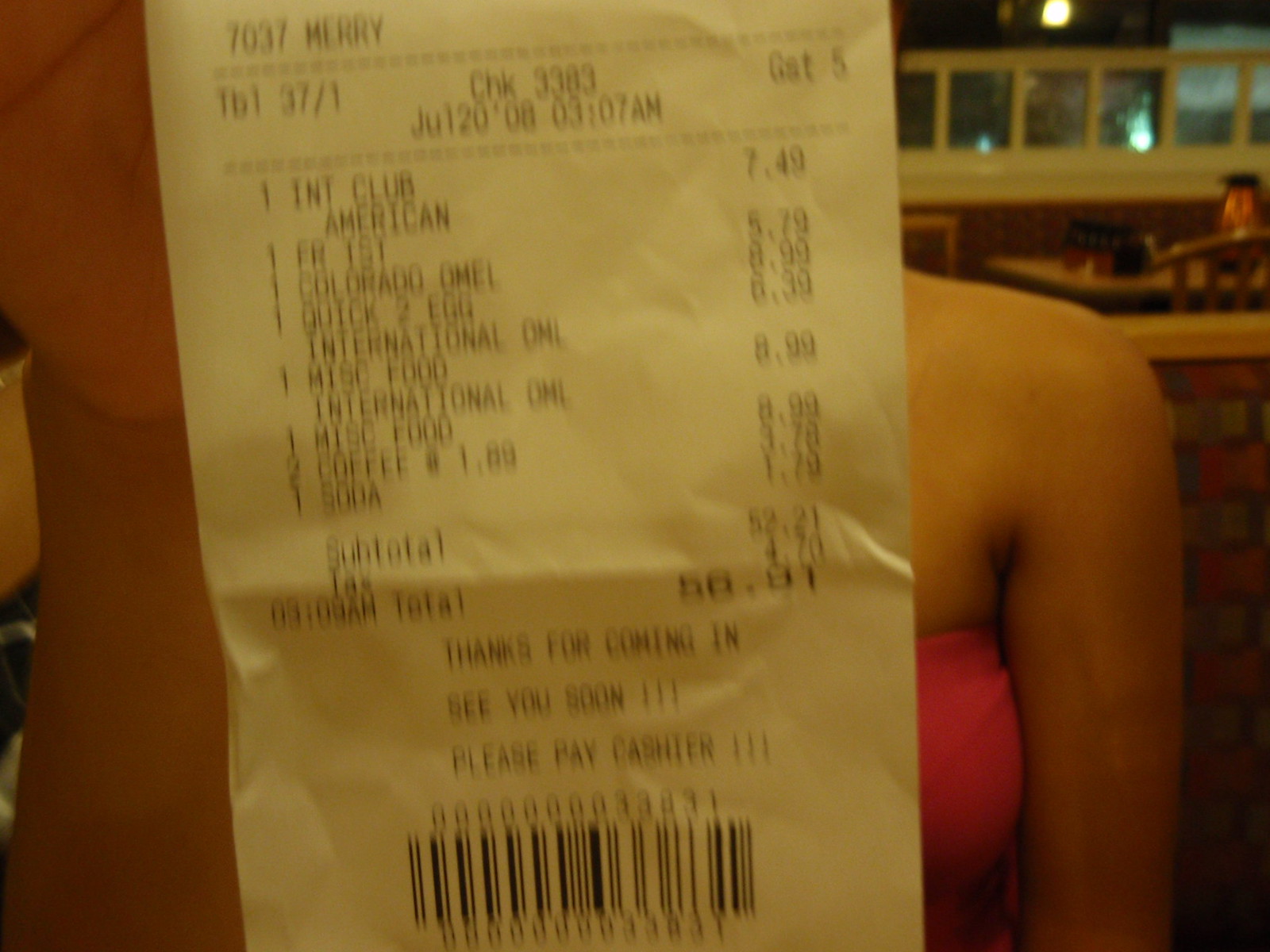The photograph captures an outdoor dining setting at night, featuring several restaurant tables and chairs beneath softly lit trees. In the background, a glass window and wooden booth with a plaid design are visible. A slender woman in a pink strapless or sleeveless top sits across from the camera, her shoulder and arm in clear view. She holds a white thermal-paper receipt up close to the camera. The receipt, dated June 20, 2008, lists items including an American Club sandwich, a Colorado Omelette, two coffees, and other miscellaneous food items, totaling $59.97. Intricate details such as a barcode and a friendly message, "Thanks for coming in, see you soon, please pay cashier," complete the scene. Another person's hand appears on the left side of the image, also holding the receipt, contributing to the intimate feel of this snapshot.